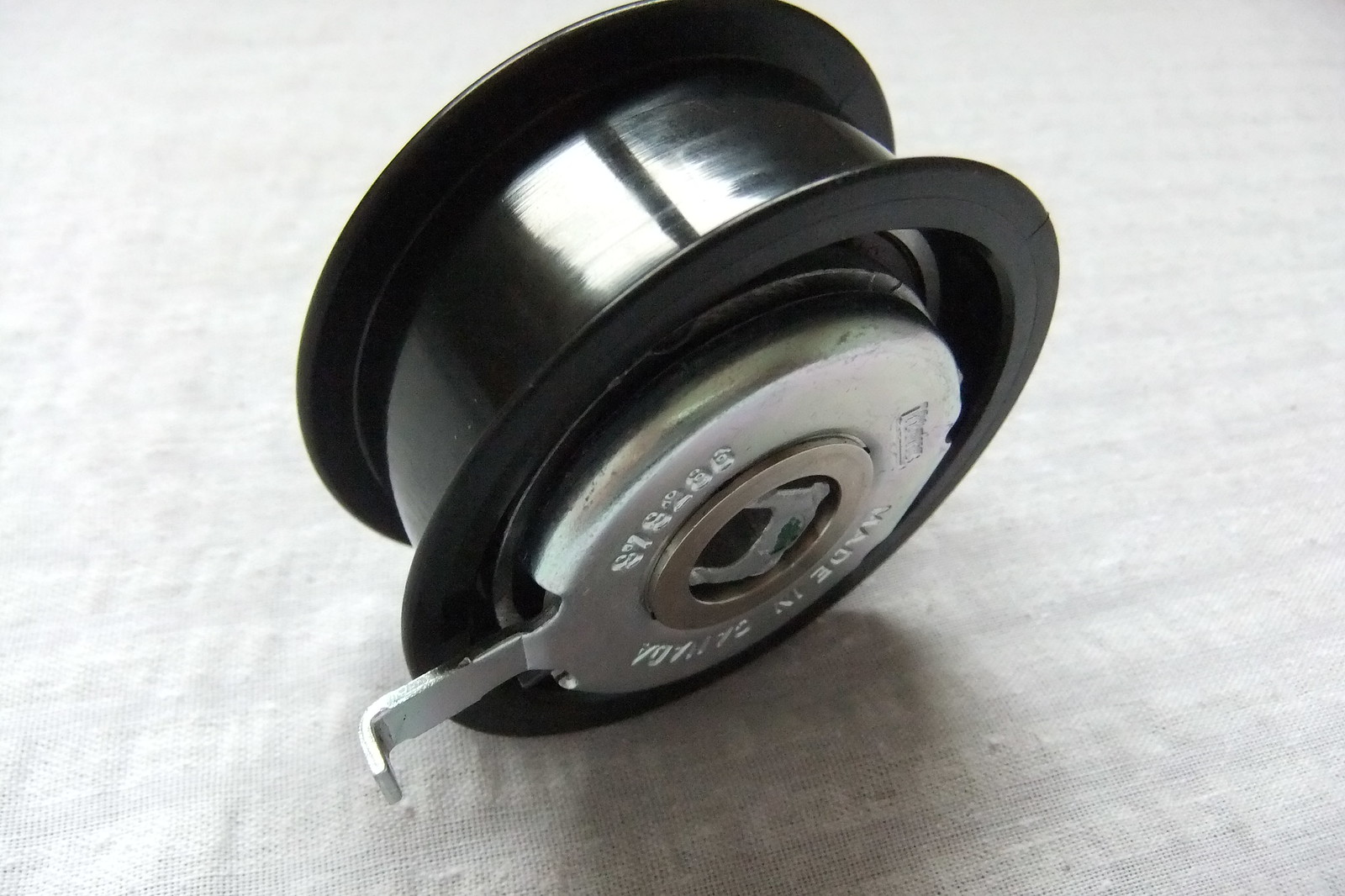The image depicts a detailed close-up of a black, wheel-like structure sitting on a white, textured surface, possibly fabric. Resembling a cylindrical bobbin or a wheel of a cart, the object features a black plastic edge with raised outer rims that make contact with the ground. The center of the wheel comprises a reflective, smooth plastic casing, within which lies a circular metal component, likely steel. This metal center includes an additional bearing and a central metal square, along with some indecipherable writing, and bears the inscription "Made in Canada." An extending metal clip runs from the central bearing to the edge, which may serve as a mechanism for stopping or starting the wheel. The intricate design and industrial look of the wheel give it the semblance of a reel for tape or a sewing machine bobbin case.